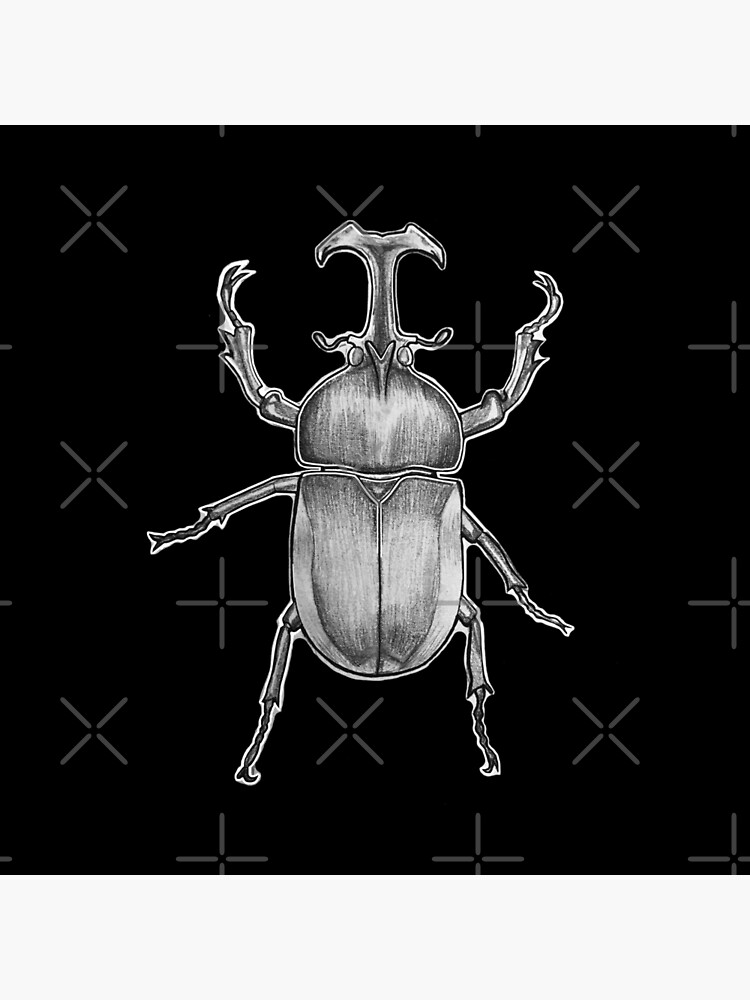This illustration features a detailed black-and-white rendering of a rhinoceros beetle, noted for its prominent horn on the head resembling a shovel. The view is from the top, showcasing the beetle's characteristic three-segment body: the head with its two spiky antennae, the thorax with three pairs of spiky legs—two emanating from the thorax and four from the abdomen. The beetle's intricate details, such as its segmented body and textured shell, are rendered in a pencil-like, monochromatic style. The background is stark black, adorned with a grid of alternating gray X's and crosses, each comprised of four lines with a void at the center, creating a pattern that highlights the beetle. The surrounding white border suggests the image might have been cropped from a larger piece, possibly for usage in a digital or print context.